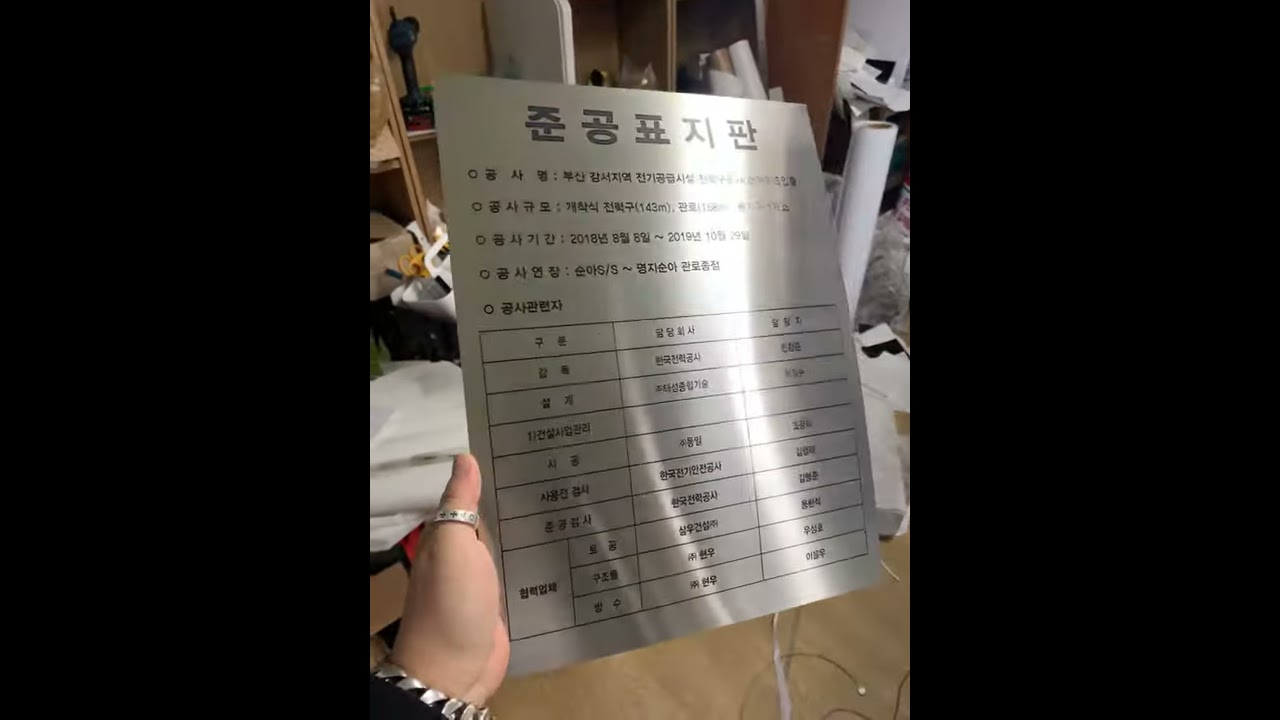This photo is a horizontally aligned rectangular image with thick black borders on both sides, focusing attention on the center. It features a close-up of a person's hand in the lower left corner, wearing a ring on their thumb and a chunky silver or gold bracelet on the wrist. The hand is holding a sheet of paper or possibly a reflective metal sign, difficult to distinguish due to glare, displaying five large black symbols at the top, likely in Korean. Below the symbols are additional text and a detailed table with columns and rows and dates including 2018 and 2019. The person’s attire includes a black shirt sleeve. The background reveals a brown tiled floor, various indistinct objects scattered around, phone charging cords, and a disorganized wooden shelf laden with miscellaneous items. The overall scene depicts a cluttered room with a clear focus on the hand-held document.